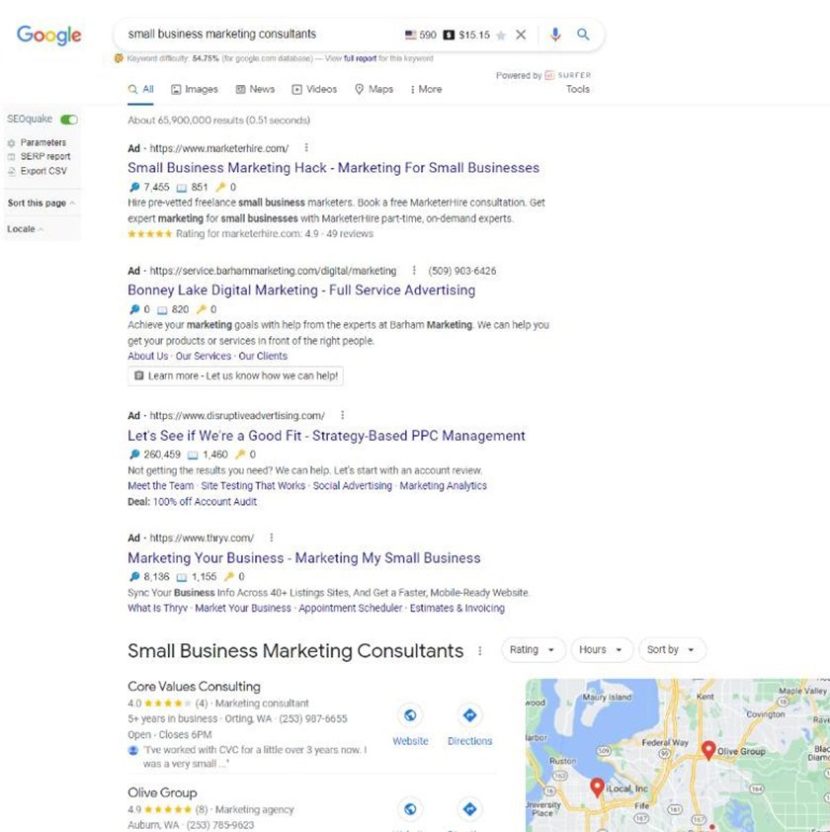This is an image showing the results of a Google search for "small business marketing consultants." The search page is presented with the familiar Google logo in its regular colors and a capital "G" on the upper left-hand side. The search results include several entries, with the first four prominently labeled as ads in bold black text. 

Further down the page, a distinct listing appears in a slightly larger font but without the ad notification. This listing is accompanied by a map highlighting relevant locations in the area of interest. Among the non-ad results, two businesses are prominently featured: Core Values Consulting, which has received a five-star rating, and Olive Group, which is rated with six stars. Both of these businesses are located relatively close to the specified search area.